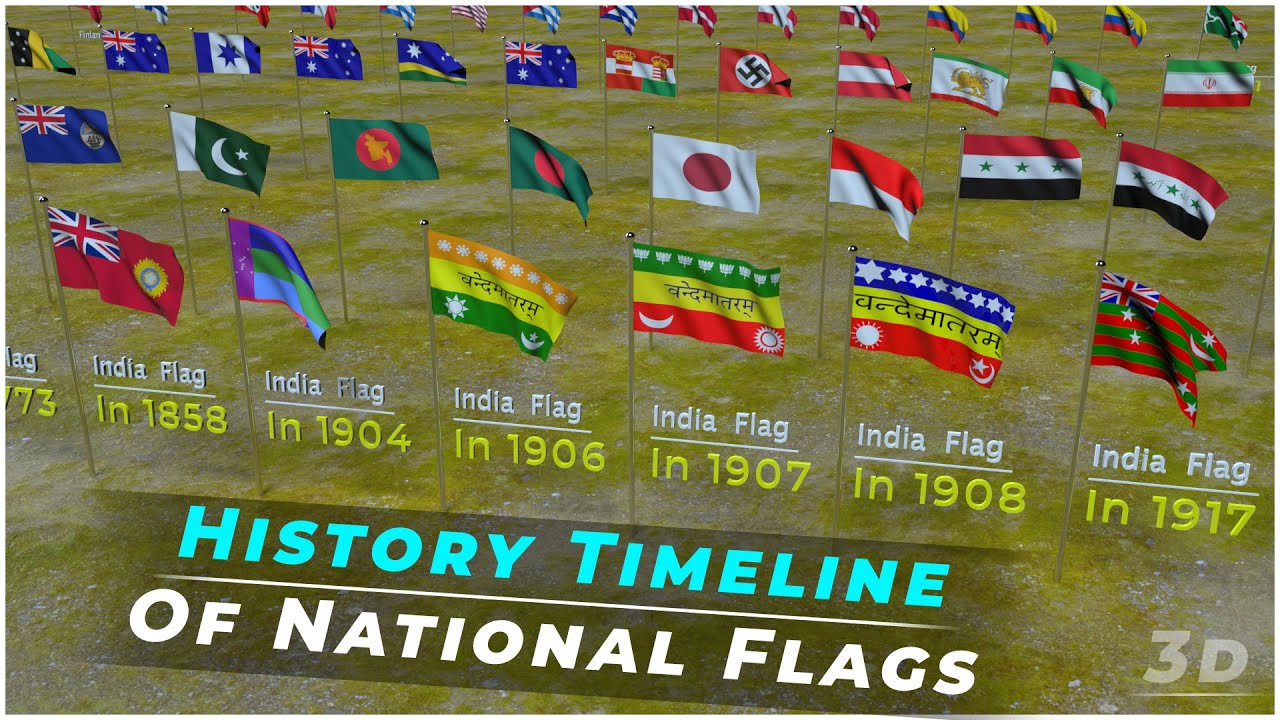The image is a highly detailed 3D render depicting a comprehensive history timeline of national flags arranged meticulously on a field. Four rows of flags span across the image, showcasing an array of national flags from various countries and eras, including the United Kingdom, Iran, Egypt, Poland, Japan, Algeria, New Zealand, Australia, France, Cuba, the United States, the Nazi flag, and the Austrian flag. Notably, the front row is entirely dedicated to Indian flags, illustrating their evolution from 1773 to 1917. Each flag's historical significance is highlighted. The bottom of the image features the text "History Timeline of National Flags" in blue and white letters, along with a 3D logo in the bottom right corner.